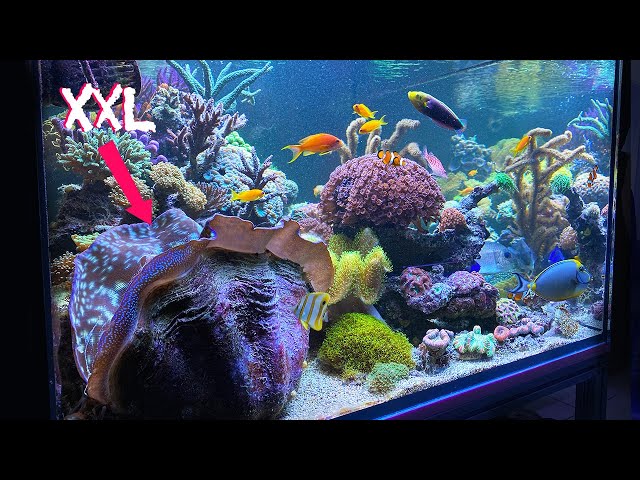The image appears to be of a vibrant tropical aquarium, showcasing a variety of brightly colored fish swimming amidst lush coral formations. The water is crystal clear, enhancing the visibility of the aquatic life within. Notably, the photograph has been edited with the letters "XXL" in the top left corner, accompanied by a pinkish-red arrow pointing down to a distinctive shell located in the lower left section of the aquarium. The scene is bustling with at least eight fish of various colors and sizes: one resembles the iconic clownfish "Nemo" from the film *Finding Nemo*, another appears to be a golden or orangish koi, a third one is purplish with a yellow face, and yet another is flat and blue, reminiscent of "Dory" from the same movie. The assortment of corals adds to the aquarium's aesthetic appeal, making it a stunning visual representation of a tropical underwater ecosystem.